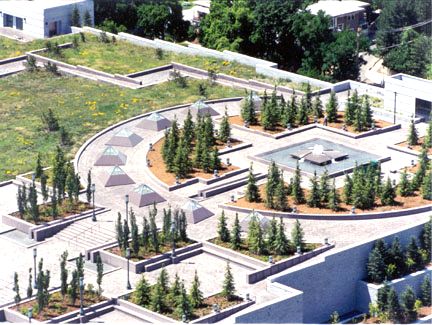This aerial photograph captures a meticulously designed garden and courtyard, likely part of a palace or museum. The top-down perspective reveals extensive detail, suggesting the photo was taken from a helicopter or airplane. Central to the composition is a square-shaped fountain, divided into four quadrants by a cross-shaped structure raised at the center, and surrounded by a pool. Encircling this water feature is a ring of neatly arranged pine trees, which is itself bordered by a larger semicircular walkway adorned with small, pyramid-shaped objects. The surrounding garden includes areas with brownish dirt and patches of grass interspersed with pine trees, seamlessly integrating the natural elements with the architectural layout. To the right, a gateway building leads into a small, square plaza that connects with the rest of the courtyard, possibly indicating an elevated or rooftop structure. The overall symmetry and the combination of natural and man-made elements make this a visually striking example of landscape design.